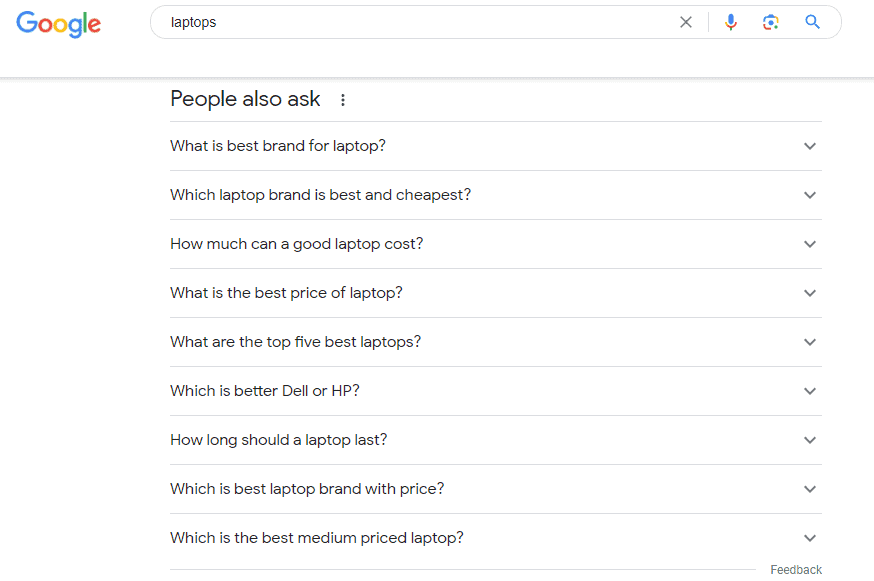This screenshot depicts a Google search results page. Dominating the top-left corner is the iconic Google logo with the first "G" and the second "G" in blue, the initial "O" and the final "E" in red, the second "O" in yellow-orange, and the "L" in green. Extending across the majority of the page is a long search bar containing the query "laptops." The background is a clean, plain white.

Below the search bar, a section titled "People also ask" showcases a list of nine frequently asked questions related to laptops:

1. What is best brand for laptop?
2. Which laptop brand is best and cheapest?
3. How much can a good laptop cost?
4. What is the best price of laptop?
5. What are the top five best laptops?
6. Which is better Dell or HP?
7. How long should a laptop last?
8. Which is best laptop brand with price?
9. Which is the best medium priced laptop?

Each question is accompanied by a small, downward-pointing arrow, indicating that tapping on them would reveal more details.

Completing the page, in the lower right corner, the word "Feedback" appears in small text. The page lacks any additional images, colors, or visual embellishments, emphasizing a minimalistic design focused strictly on text-based content and user queries.